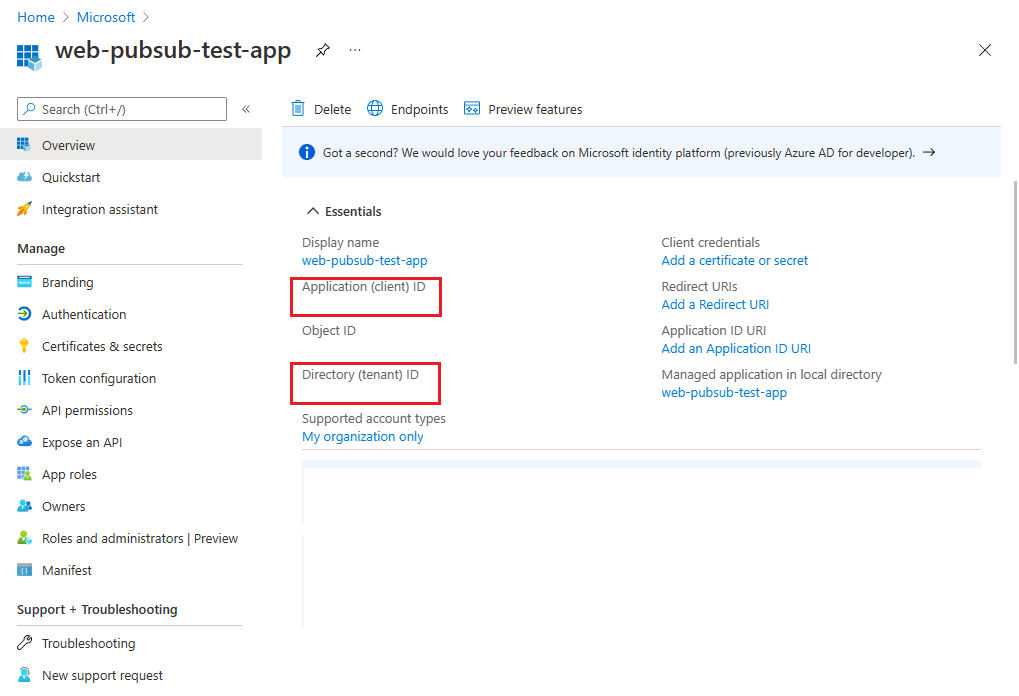**Captured Image Description:**

The image appears to be a screenshot from a website, presented against a white backdrop. The layout is organized with several labeled icons and navigation elements:

- **Top Navigation:** On the top left corner, the text "Home" in blue is accompanied by a gray outlined arrow pointing to the right. Next to it, "Microsoft" is similarly blue with a right-pointing gray arrow.

- **Main Content Area:**
  - **Title and Identification:** Below the navigation, there is a blue box composed of nine smaller squares (three rows of three). In front of the bottom right corner of this box, there's a lighter blue square. To the right, the text "web-hubsub, PUBSUB-test-app" appears in black, followed by a black thumbtack icon and three black dots. On the far right of the page, there's a black "X".
  - **Search Bar:** Under the title, the term "web-hubsub test app" is repeated with a search bar beneath. The search bar includes the word "search" in black, a double arrow facing left, a blue garbage can icon labeled "delete" in black, a blue globe icon labeled "end point" in black, and a blue box labeled "preview features" in black.

- **Left Pane Navigation:**
  - Various sections are listed vertically, alongside corresponding icons:
    - A blue box next to the word "overview".
    - A blue cloud labeled "quick start".
    - A yellow rocket ship icon next to "integration assistant".
    - "Manage" in black text. 
    - A list of functional sections with respective icons, including:
      - A blue box with the term "branding".
      - A blue semi-circle with a green arrow labeled "authentication".
      - A yellow key for "certificates and secrets".
      - Three blue bars for "token configuration".
      - A greenish semi-circle for "API permissions".
      - A blue cloud labeled "expose an API".
      - A blue box made up of nine small squares labeled "app roles".
      - An indeterminate blue logo for "owners".
      - A green person icon for "roles and administrators".
      - A vertical line followed by "preview".
      - A blue box labeled "manifest".
      - "Support + troubleshooting" section followed by:
        - A wrench icon and "troubleshooting".
        - A blue person icon and "new support request".

- **Granular Details (Top Section):**
  - Below “delete endpoints and preview features,” there's a blue bar featuring a darker blue circle with an "I" inside, with the text: "Got a second? We would love your feedback on Microsoft Identity Platform (previously Azure AD for developers)" in black. 
  - "Essentials" section:
    - "Display name" followed by "web PubSub test app" in blue.
    - "Application (client ID)", "Object ID", and "Directory (tenant ID)".
    - "Support account types" followed by "My organization only" in blue and "client credentials".
    - "Add a certificate or secret" in blue.
    - "Redirect URIs" in black, followed by "Add a redirect URI" in blue.
    - "Application ID URI" with the option to "Add an application ID URI" in blue.
    - "Managed application in local directory" followed by "web-PubSub-test-app" in blue.

- **Informational Boxes:**
  - **Announcements:**
    - A blue bar with a blue circle and white "I" containing the message: "Welcome to the new and improved app registrations. Looking to learn how it's changed from app registrations (legacy)?" followed by "Learn more" in blue.
    - Below, another blue box with a dark blue circle and white "I" communicates the message: "Starting June 30th, 2020, we will no longer add any new features to Azure Active Directory authentication library (ADAL) and Azure AD Graph. We will continue to provide technical support and security updates but will no longer provide feature updates. Applications will need to be upgraded to Microsoft Authentication Library (MSAL) and Microsoft Graph." This is followed by "Learn more" in blue.
    - A "Get started" link underlined in blue, with a "Documentation" link to the right.

This detailed layout provides a comprehensive overview of the different sections and functionalities available in the application interface captured in the image.